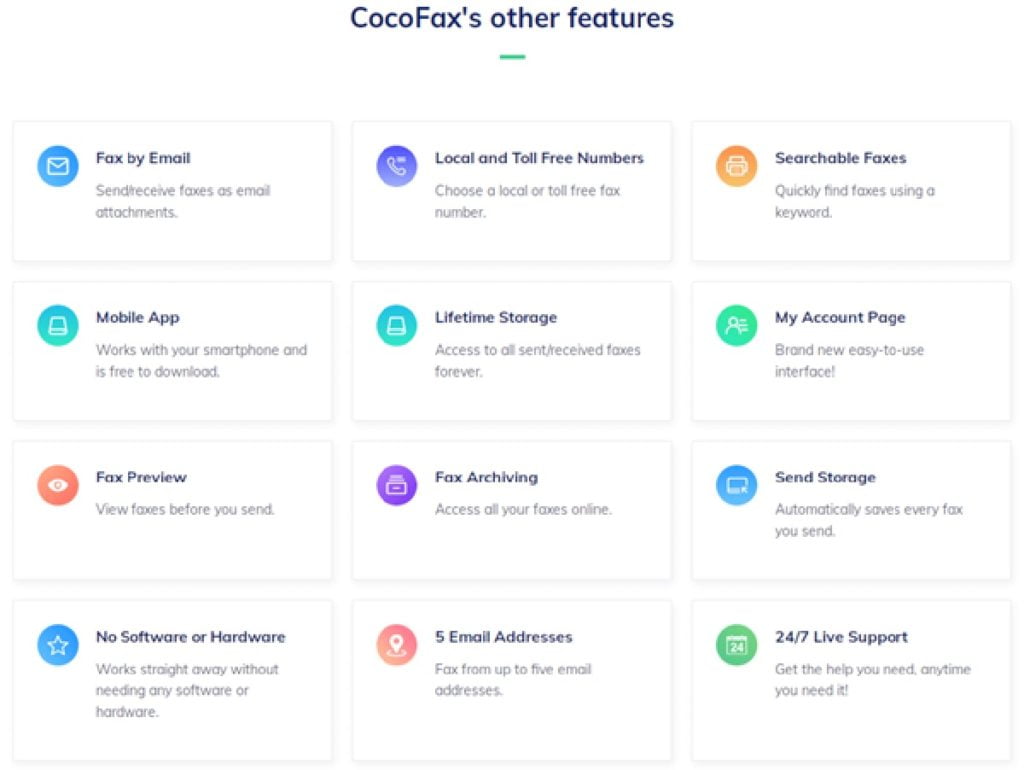The screenshot displays a collection of twelve different menu options, arranged in a three-by-four grid from left to right. 

- **Top Row:**
  - **Fax by Email:** Features a blue image of an envelope, with the description "Send/receive faxes as email attachments."
  - **Local and Toll-Free Numbers:** Displays a purple phone icon and notes "Please choose a local or toll-free fax number."
  - **Searchable Faxes:** An orange printer icon accompanies the text "Quickly find faxes using a keyword."

- **Second Row:**
  - **Mobile App:** Shows a blue computer and mentions "Works with your smartphone and is free to download."
  - **Lifetime Storage:** Features the same blue computer icon, stating "Access to all sent/received faxes forever."
  - **My Account Page:** Highlights a green person icon with the description "Brand-new easy-to-use interface."

- **Third Row:**
  - **Fax Preview:** An orange eye icon allows you to "View faxes before you send."
  - **Fax Archiving:** Displays a purple printer icon with the text "Access all of your faxes online."
  - **Sent Storage:** Shows a blurred blue image and notes "Automatically saves every fax you send."

- **Bottom Row:**
  - **No Software or Hardware:** Features a blue star icon, indicating "Works straight away without needing any software or hardware."
  - **Five Email Addresses:** Depicts a reddish-orange location icon, stating "Fax from up to five email addresses."
  - **24/7 Live Support:** A green calendar icon signifies "Get the help you need anytime you need it."

Each menu option is encased in a white box with black text for clear readability.